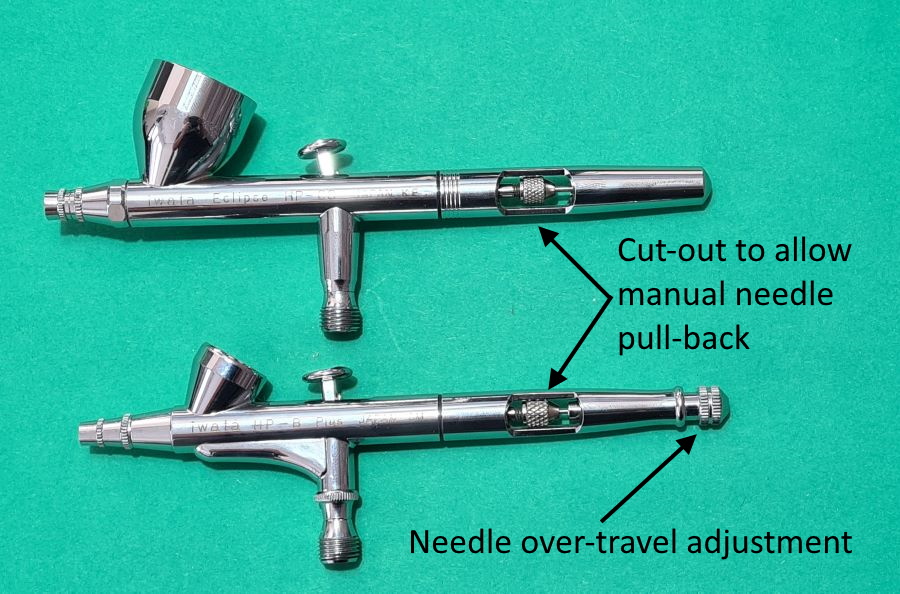The image features a pair of polished silver devices horizontally aligned in the center of a teal green background, which occupy a horizontally aligned rectangular space. Both devices, resembling instruments used with air compressors or tire gauges, have several distinctive features and are slightly different in size. The devices have narrow, cylindrical shapes with slightly pointed tips on the left side, possibly for connecting to an inflation mechanism. 

Each device has multiple components, including tubes with various protrusions like sockets, pins, levers, and threaded sections, which appear to allow for different functions and attachments. Notably, the center sections of both devices have cut-out areas with text and arrows pointing to them, indicating that these sections are designed to "cut out to allow manual needle pullback." Additionally, the bottom device features an adjustment area highlighted by a separate arrow with accompanying text that reads "needle over travel adjustment," pointing to a small, round adjustment wheel near the tip.